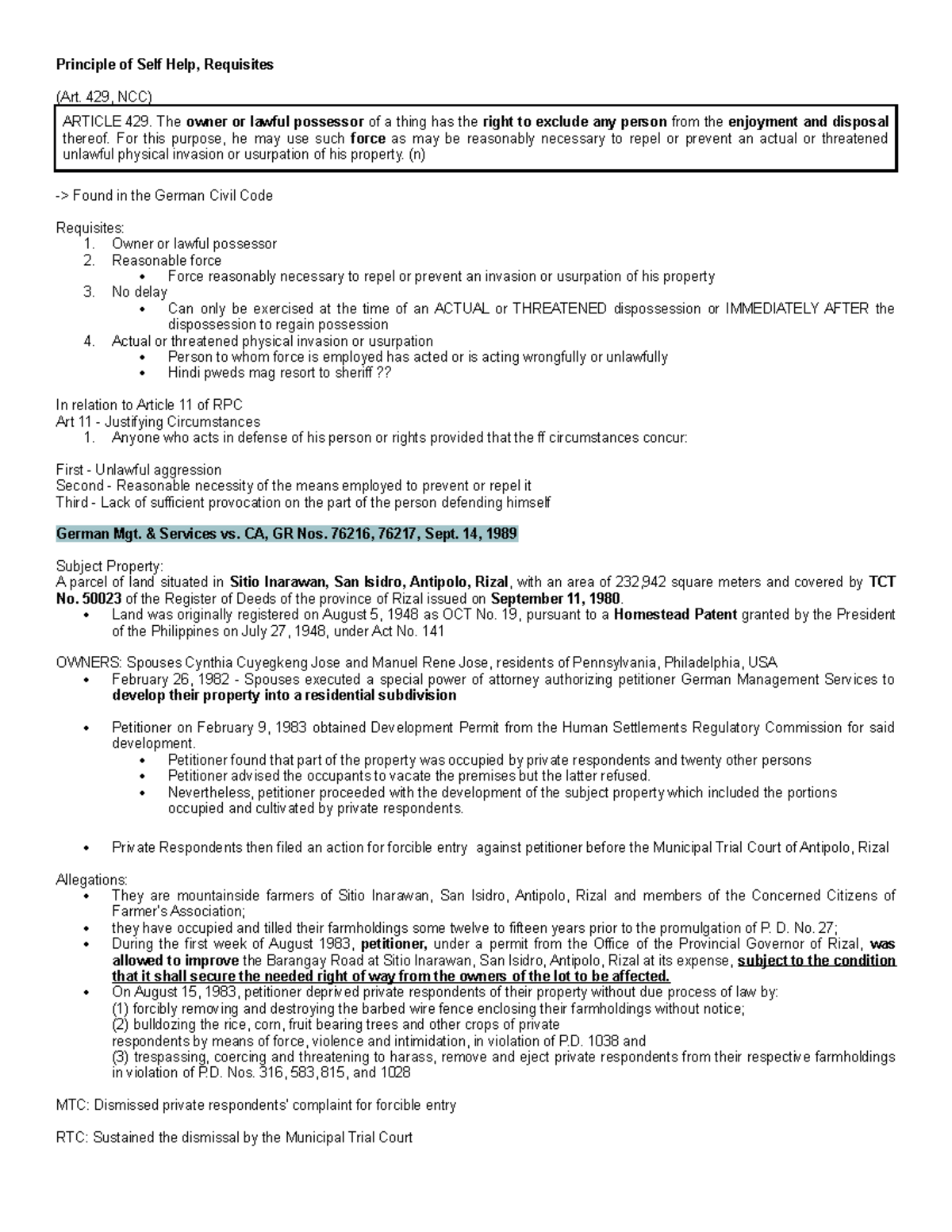**Principle of Self-Help Requisites**

This screenshot prominently features the bolded text "Principle of Self-Help Requisites" in the top left corner. Below this, a black rectangular box highlights Article 429, which states, "The owner or lawful possessor of a thing has the right to exclude any person from enjoyment and disposal thereof. For this purpose, he may use force as may reasonably necessary to repel or prevent an actual or threatened unlawful physical invasion or usurpation of this property." This article is found in the German Civil Code.

The content then lists some requisites to exercise this right, including:
- Owner or lawful possessor
- Reasonable force
- No delay
- Actual or threatened physical invasion or usurpation

There is also information related to Article 11 of the Revised Penal Code (RPC), marked by blue-highlighted text. Additionally, there are references to MGT and services risks, indicated by the Compound Annual Growth Rate (CAGR) numbers, and the date September 14, 1989.

The subject property, its owners, and their situations are detailed with bullet points:
- Main bullet points regarding the property
- Allegations which enumerate four specific points 

Finally, it mentions MTC and RTC, likely referring to Municipal Trial Court and Regional Trial Court respectively.